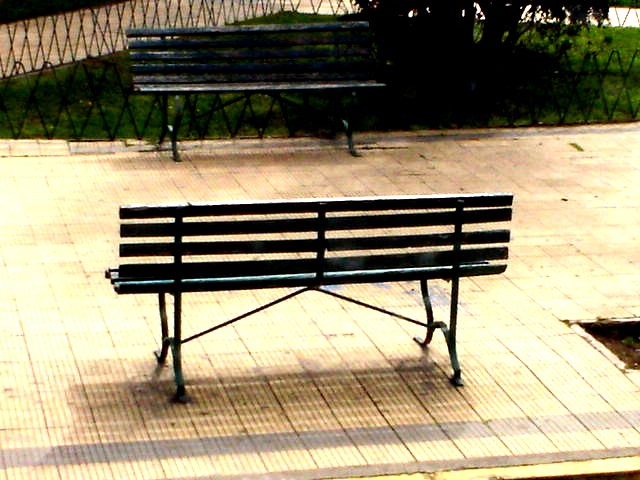The photograph showcases two park-style benches facing each other on a patterned tiled walkway. The benches are painted a dark color, possibly black or deep green, and their surfaces appear worn or mottled, suggesting they may be made of metal with a potential verdigris finish, giving them a combination of dark brown and green hues. The nearest bench is seen from the back, while the farther bench faces the viewer. Both benches feature slatted seats that curve from the seat base up to their backs, supported by wrought iron legs with angled support struts centered under the benches. 

The walkway between the benches is golden beige in color, bordered by faint red grid-patterned tiles, and segmented by strips of pale yellow and grayish sections. Beyond the distant bench, there is a short metal fence composed of a series of black diamond-shaped outlines formed by crossed metal bars. This fence delineates a green space with lush grass and at least one visible tree, with additional trees casting shadows across the scene. Another beige stone walkway with a black metallic fence rings seen in the upper left corner adds further structure to the setting, enhancing the organized yet natural aesthetic of the park area.